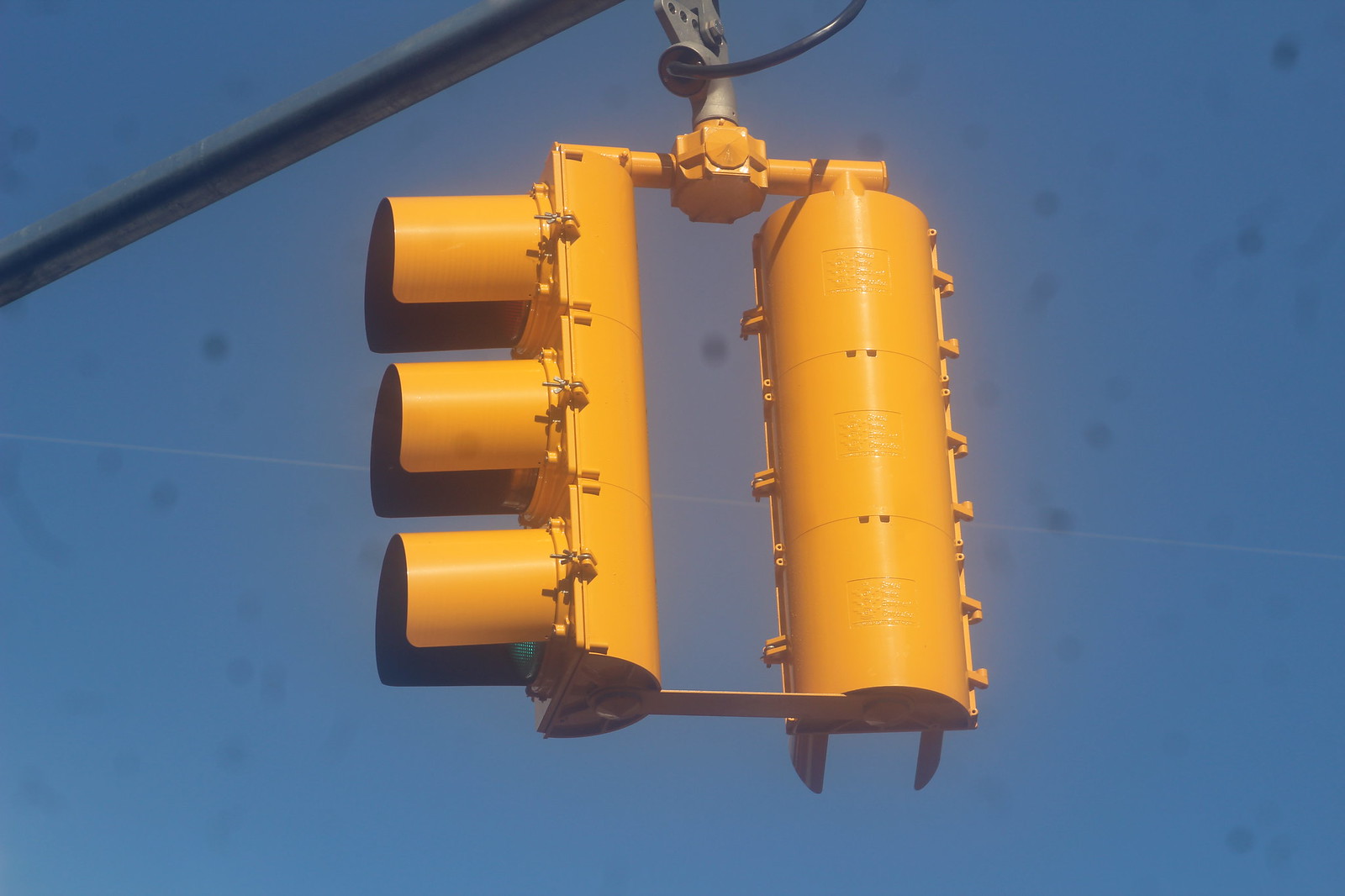This photograph captures a pair of yellow traffic signals hanging from a horizontal silver pole against a clear blue sky. The setup includes two traffic lights connected by a yellow bracket. The traffic light on the right, seen from the rear, is a round half-cylinder with two sets of square holes on its back. The traffic light on the left is depicted in profile, featuring three cylindrical shields, or hoods, extending perpendicularly from the flat face of its half-cylinder frame to prevent light misreading from other angles. Additionally, there is a gray hinge and a black wire visible at the top where the traffic signals attach to the supporting pole. The image is marred by gray discoloration spots that may be due to a dirty camera lens, a dirty window, or possibly spots on printed film. The scene is framed against a bright, uninterrupted blue sky, with some white streaks and scattered gray dots throughout.